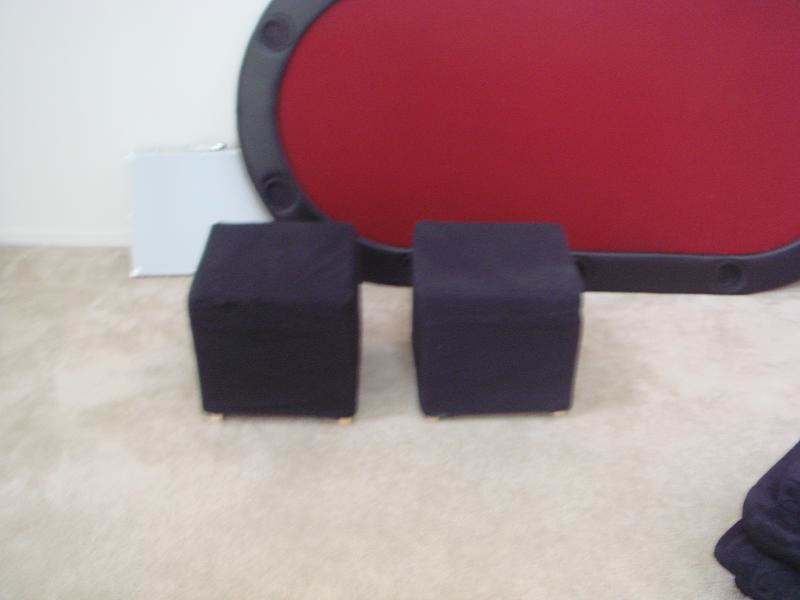The image depicts a basement setting with a light beige carpeted floor. Prominently, there is a red, oval-shaped poker table with a black leather border featuring circular drink holders, lying on its side against a white wall. Nearby, a silver poker set case is visible, possibly holding chips and cards. In front of these, two small navy blue ottomans with beige wooden seats and light-colored feet rest side by side. The ottomans are cube-shaped and covered in a black cloth, appearing more as decorative pieces than functional seats. Additionally, in the bottom right corner, there are a couple of black, velour-textured cushions partially visible. The image is very blurry, making finer details hard to discern.